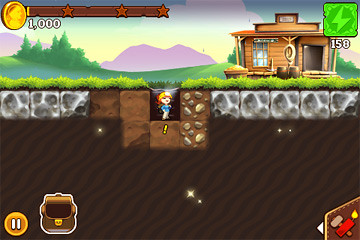A screenshot of a mobile game showcasing a detailed user interface is presented. In the upper right-hand corner, a green lightning bolt icon accompanied by the number '158' indicates the remaining moves or energy. The upper left features a progress bar with three brown stars and a coin icon labeled '1000,' suggesting this bar fills up as coins are collected. Positioned in the bottom left are a pause button next to a backpack icon, while the bottom right includes a hammer and a dynamite icon, implying tools for digging. The central section of the image focuses on a character, a woman, positioned on grassy terrain beside a small shack, with dirt and rocks stretching beneath her, indicating the objective involves excavation into the ground.